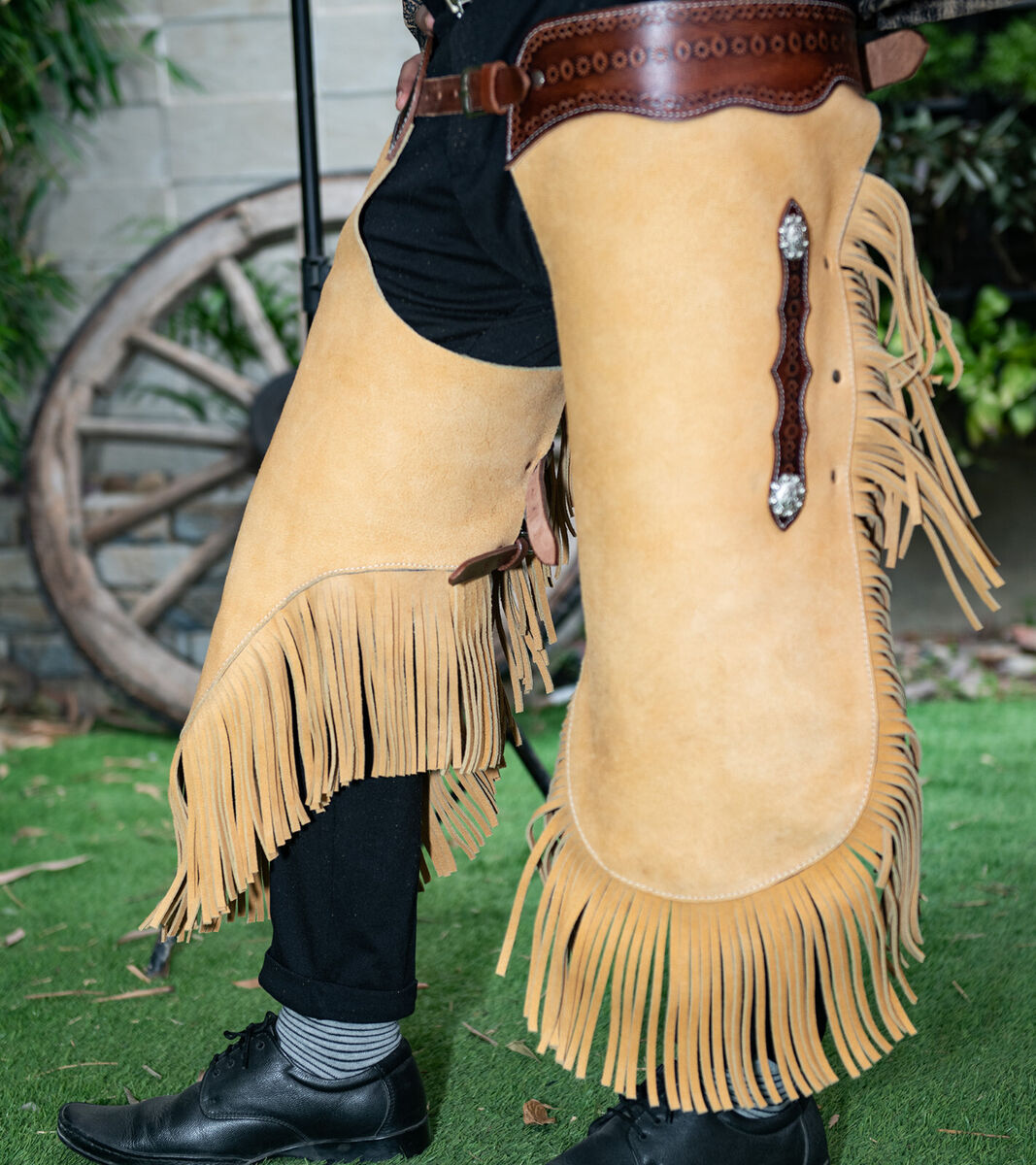The image depicts the lower half of a person dressed in ornate cowboy attire. The focal point includes a pair of camel-colored leather chaps, adorned with fringe detailing along the edges. These chaps feature inset patches of darker brown leather, each embellished with two decorative silver emblems. The person, who might be a woman based on the small size of the feet, wears black pants underneath the chaps, which also show lighter brown leather belting around the waist. The chaps are designed to be longer in the front than in the back. Completing the outfit are black, pointy shoes paired with gray and black striped socks. The setting appears to be an artificial environment resembling the outdoors, featuring green turf and a background with a gray brick wall and a wooden wagon wheel leaning against it, which adds to the western theme.